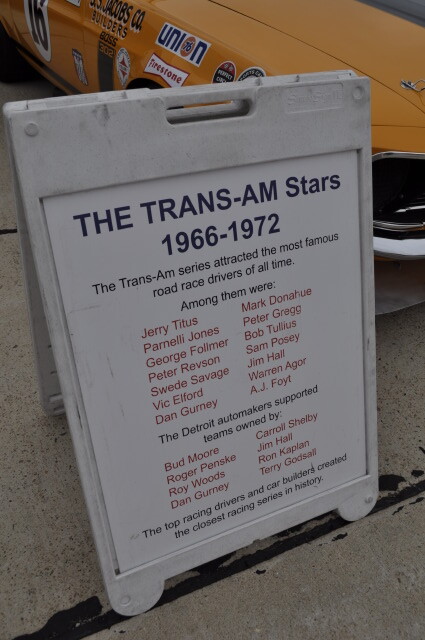In the image, there is a prominently placed white plastic sign on the ground at what appears to be an auto show or convention. The top of the sign features the title "The Trans Am Stars 1966-1972" in navy blue lettering. Below this, in black font, it states, "The Trans Am series attracted the most famous road race drivers of all time." The sign then lists 14 renowned drivers in red font across two columns: Jerry Titus, Parnelli Jones, George Follmer, Peter Revson, Swede Savage, Vic Alford, and Dan Gurney on the left, with Mark Donahue, Peter Gregg, Bob Tullius, Sam Posey, Jim Hall, Warren Agor, and A.J. Foyt on the right.

Further down, in black text, the sign explains that "The Detroit automakers supported teams owned by," followed by another list of notable figures in red font: Bud Moore, Roger Penske, Roy Woods, and Dan Gurney on the left, and Carroll Shelby, Jim Hall, Ron Kaplan, and Terry Godsall on the right. At the very bottom, the sign concludes that these top racing drivers and car builders "created the closest racing series in history."

In the background, partially visible behind the sign, is the lower half of an orange race car with several sponsor stickers, including noticeable ones for Union and Firestone. The car also features a distinctive number 16 within a white circle.